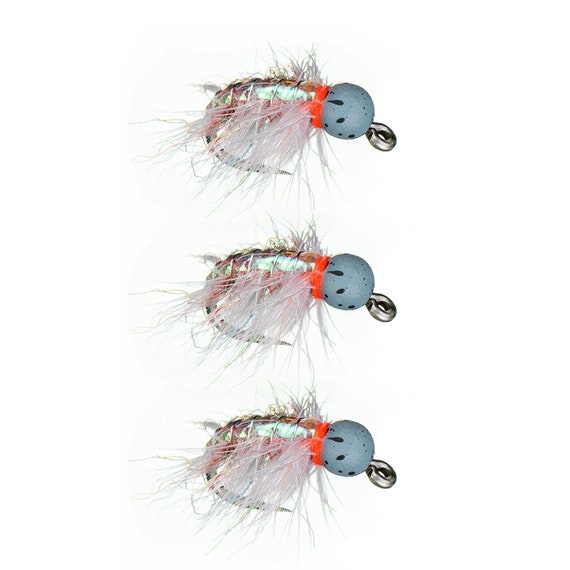This photograph features three identical fishing lures, arranged vertically against a white background. Each lure consists of a small, silver hook at the top for threading a fishing line. Below this, a light blue sphere is adorned with dark blue splotches. This sphere is followed by a small, fluorescent orange-red band, referred to in one caption as a "neck". Each lure's hook is decorated with messy, white feathers, creating an impression of plastic fibers or thin threads. The hooks themselves are sharp and metallic, with red detailing extending towards the bottom. Despite slight variations in descriptions, all lures are consistently represented, each an exact replica of the other two, suggesting possible use of digital manipulation.